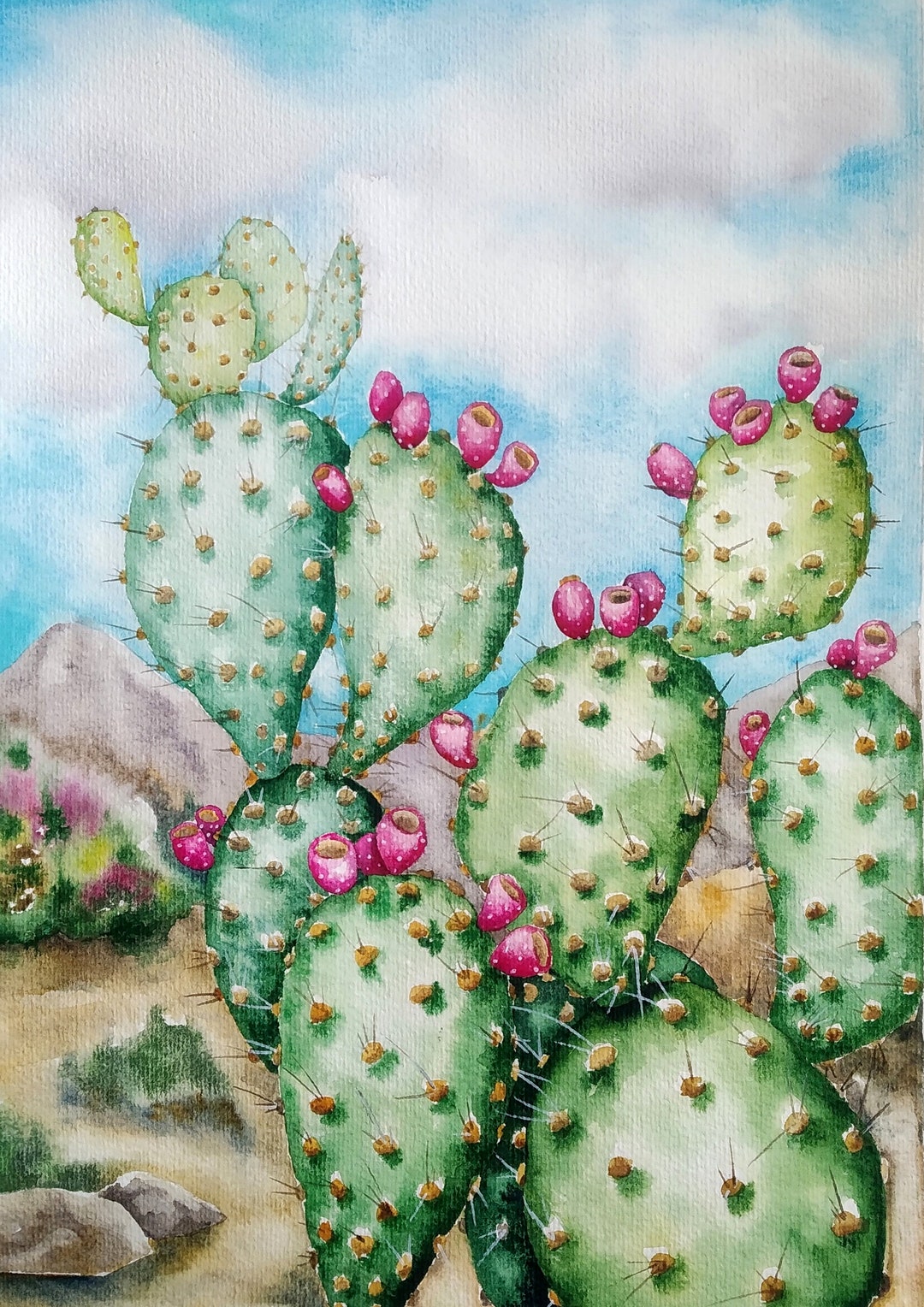The watercolor painting depicts a vibrant desert scene centered on a prickly pear cactus. The cactus, composed of green teardrop-shaped paddles connected in a layered arrangement, features numerous brown thorn clusters and vivid pink flowers adorning several of its paddles. The detailed, whimsical color palette emphasizes the edges of the plant, lending a lively and almost cartoonish quality to the cactus. In the foreground, the sandy, tan-colored desert ground is dotted with occasional patches of greenery and small rocks. The background reveals a low, light brown mountain range under a sky of soft blue with white and gray clouds, adding depth to the composition. The overall scene is both detailed and richly colored, capturing the essence of a lively desert landscape.